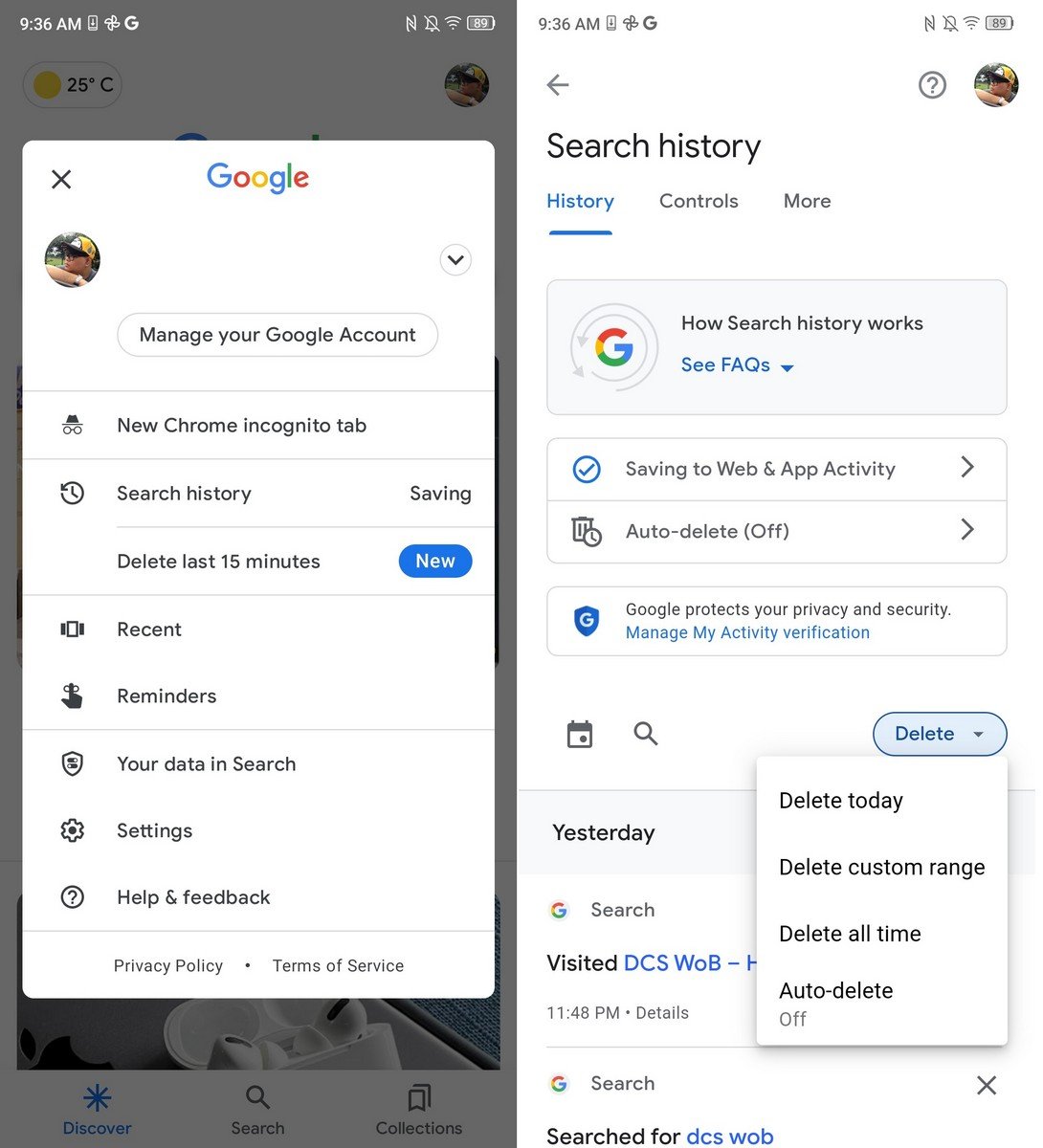**Detailed Caption:**

In this dual-image set, the first image features a smartphone screen displaying an application, specifically a Google account settings menu. The status bar at the top right corner shows it is 9:36 AM, alongside icons indicating the presence of Wi-Fi and a partially charged battery. The prominent feature of the image is a pop-up menu within the Google application, filling approximately 75% of the screen. The menu contains several options: "Manage your Google Account," "New Chrome Incognito Tab," "Search History," "Saving," "Delete last 15 minutes" (notably marked as a new feature), "Recent," "Reminders," "Your data in Search," "Settings," "Help and feedback," "Privacy Policy," and "Terms of Service." The underlying application interface is partially visible but largely obscured by this menu.

The second image appears to follow from the user's selection of "Search History" from the first image's menu, unveiling the search history management screen. Here, "History" is highlighted as the active tab, with additional tabs for "Controls" and "More." The screen provides insights and options such as "How search history works," "FAQs," "Saving to Web and App Activity," and "Auto-delete (off)." It emphasizes Google’s efforts in "Protected privacy and security management" and includes activity verification details. A prominently highlighted button labeled "Delete" has been interacted with, presenting users with options to "Delete today," "Delete custom range," "Delete all time," and "Auto-delete." In the background, a section labeled "Yesterday" lists recent search activity, including a search for "DCSWOB," which is reflected in the visited search results. 

This comprehensive depiction highlights the intricate details of managing and deleting search history within a Google account on a mobile device.